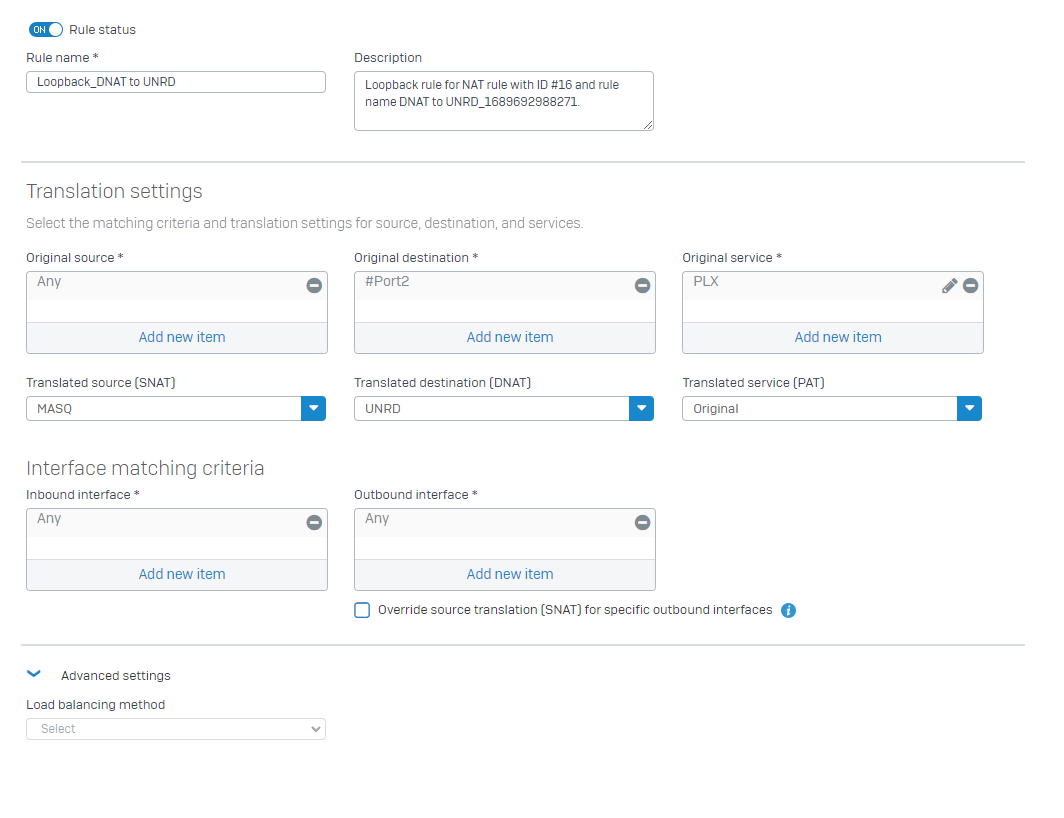This image appears to be a screenshot from a computer screen, featuring a user interface related to network configuration, specifically dealing with Network Address Translation (NAT) rules. The interface has a white background with various sections and gray text and boxes.

At the top of the image, there is a toggle switch labeled "Rule Status," which is currently in the "On" position. Directly beneath this toggle, there's a label that reads "Rule Name," next to a text box that says "loopback_DNAT_to_UNRD." 

To the right, there's a description box containing the text: "Loopback rule for NAT rule with ID number 16 and rule name in. DNAT to UNRD_168969288271."

A gray line separates this section from the next, which is labeled "Translation Settings." Below this heading is a detailed instruction: "Select the matching criteria and translation settings for source, destination, and services."

There are three horizontally aligned boxes, each labeled accordingly:
1. "Original Source" - with the content displayed as "Any"
2. "Original Destination" - with the content displayed as "Number port 2"
3. "Original Service" - with the content displayed as "PLX"

Below these boxes are three drop-down menus for translation settings:
1. "Translated Source (SNAT)" - with "MASQ" selected
2. "Translated Destination (DNAT)" - with "UNRD" selected
3. "Translated Service (PAT)" - with "Original" selected

Further down, there's a section titled "Interface Matching Criteria," which includes:
1. "Inbound Interface" - displaying "Any"
2. "Outbound Interface" - also displaying "Any"

At the very bottom of the image, there's a section labeled "Advanced Settings" featuring a drop-down menu for "Load Balancing Method."